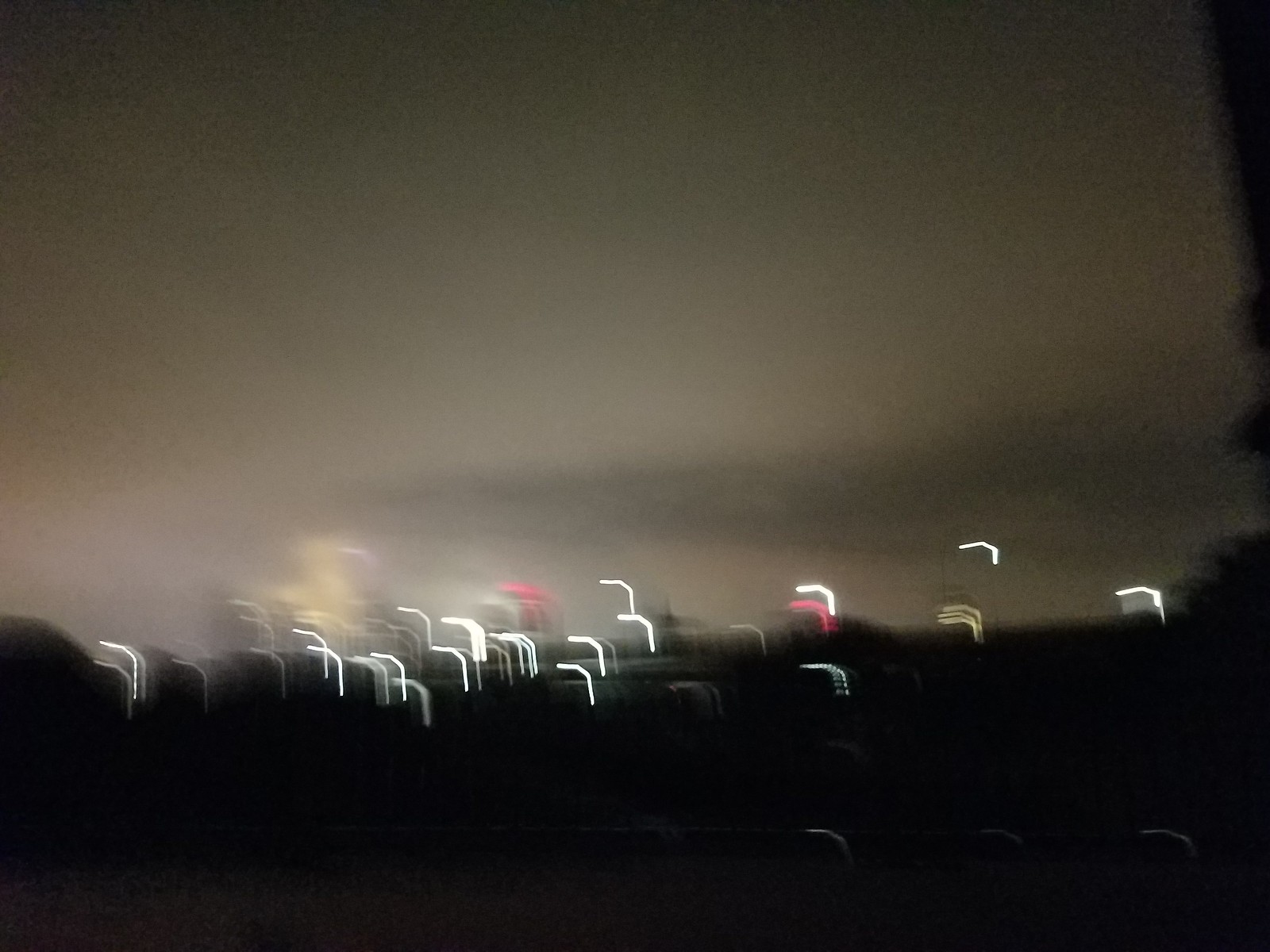The image depicts a very blurry and out-of-focus scene taken at night, likely in a graveyard. The bottom part of the image is completely dark, almost black. Above this dark area, a range of lighter, grayish tones can be seen, indicating a dark, cloudy sky. The scene features several headstones, or at least their silhouettes, which are very blurry. These headstones are outlined with various colored lines, primarily white, yellow, and pink, making shapes that resemble upside-down, backwards-facing Ls. This visual might be enhanced by some reflections or lighting distortions, possibly from something metallic that’s catching and refracting light. Additionally, some blurry lights in the image appear to form bent, almost scraggly shapes reminiscent of the number seven, in white, yellow, and a few red hues. These lights contribute to the overall eerie and indistinct appearance of the graveyard at night. On the right side, there is a hint of trees further adding to the outdoor, nighttime setting.